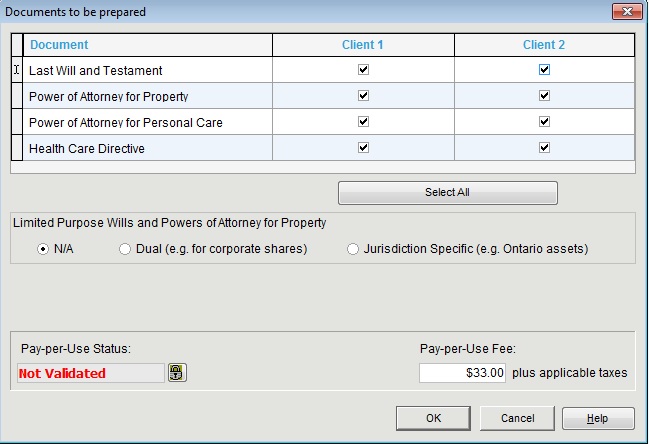A tense and dramatic moment unfolds in the dimly lit room as a concerned individual anxiously checks on another's supplies, including food, water, and medicine. The urgency in their voice escalates as they discover Octavia's unexpected absence, realizing she is hidden in the ceiling. With emotions running high, a dire warning is issued about potential consequences should anything happen to her. The scene hits a crescendo as Bellamy is forcefully confronted amidst the chaos, with urgent demands to secure necessary medication, highlighting the desperate situation and intense atmosphere permeating the room.